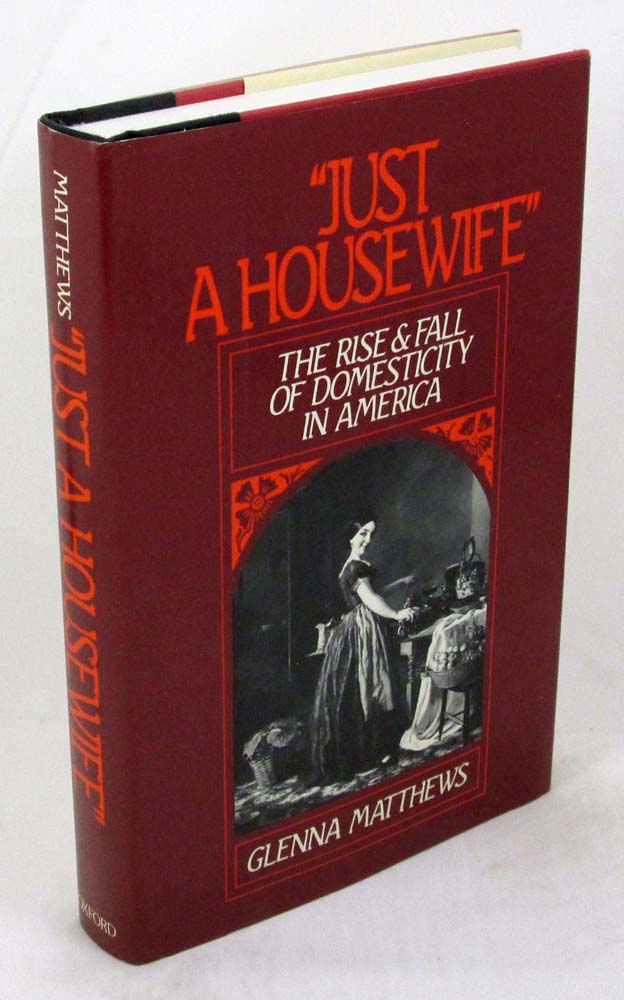The image showcases a hardcover book, entitled "Just a Housewife: The Rise and Fall of Domesticity in America" by Glenna Matthews. The book, standing upright, features a dark red dust jacket with the title in bold red text at the top. Below the title, centered within a vertical rectangle, is a black and white photograph of a woman from the early to mid-20th century. She is dressed in a long, flowery dress and appears to be engaged in domestic chores by a sewing machine, smiling towards the camera. The photograph is evocative of a bygone era, perhaps from the 30s or 40s. Above the photograph in white letters is the subtitle, "The Rise and Fall of Domesticity in America," with the author's name in white at the bottom. The background of the image is an abstract gray, giving no additional context, and the book is resting on a floor with a slight shadow indicating the camera's angle.